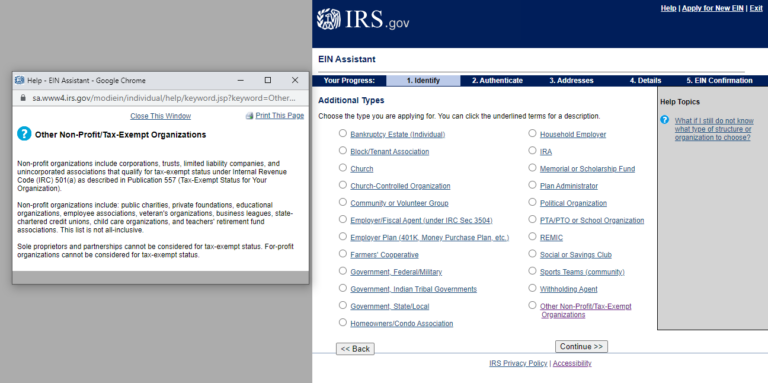Screenshot Description: 

The screenshot features a user interface with a gray background and a white pop-up box in the middle. The interface appears to be part of a website, likely the IRS website. The top of the pop-up box contains two blue links: "Close this window" and "Print this page." 

Below these links, there is a section titled "Other Non-Profit Tax Exempt Organizations," marked by a blue circle with a white question mark inside. The text details that non-profit organizations can include corporations, trusts, limited liability companies, and unincorporated associations. These entities qualify for tax-exempt status under Internal Revenue Code (IRC) Section 501(a), as further described in Publication 557, "Tax Exempt Status for Your Organization." Additional information is also hinted at but not fully visible.

In the main content area, the IRS website navigation is visible, labeled "irs.gov EIN Assistant." The navigation steps for the process are outlined and include five distinct phases: 
1. Identity (highlighted in light blue)
2. Authenticate 
3. Addresses 
4. Details 
5. EIN Confirmation

The current step, "Identity," is highlighted in light blue, indicating the user's progress in filling out the form. At the bottom of the pop-up box, there is a section labeled "Additional Types: Choose a type you are applying for. You can click the undefined terms for a description."

Overall, the screenshot captures the detailed process of applying for an Employer Identification Number (EIN) for non-profit tax-exempt organizations via the IRS's online assistant tool.